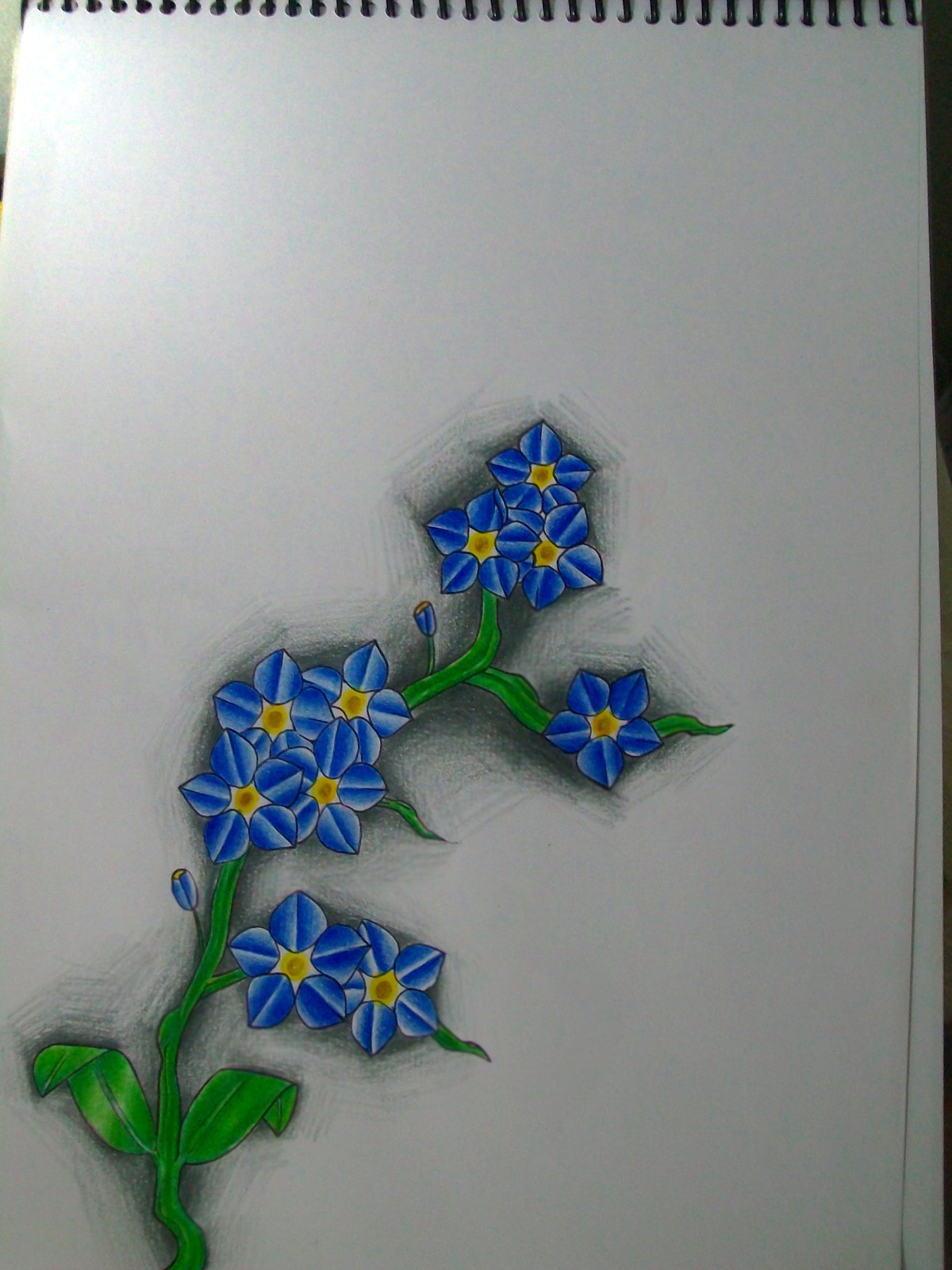In the image, there is a spiral notebook positioned horizontally with its spiral binding running across the top edge. A small section of a brown table is visible underneath the notebook. Towards the bottom left corner, a green stem ascends, adorned with two large green leaves that are slightly folded over. As you follow the stem upwards, two charming blue flowers with yellow centers appear. Continuing along the stem, four more delicate blue flowers, each with a yellow center, are visible. A tiny leaf protrudes from the stem, which then splits into two branches. One branch bears a single blue flower, while the other branch supports three blue flowers. These dainty blossoms also feature tiny white lines within their petals, adding to their intricate beauty.